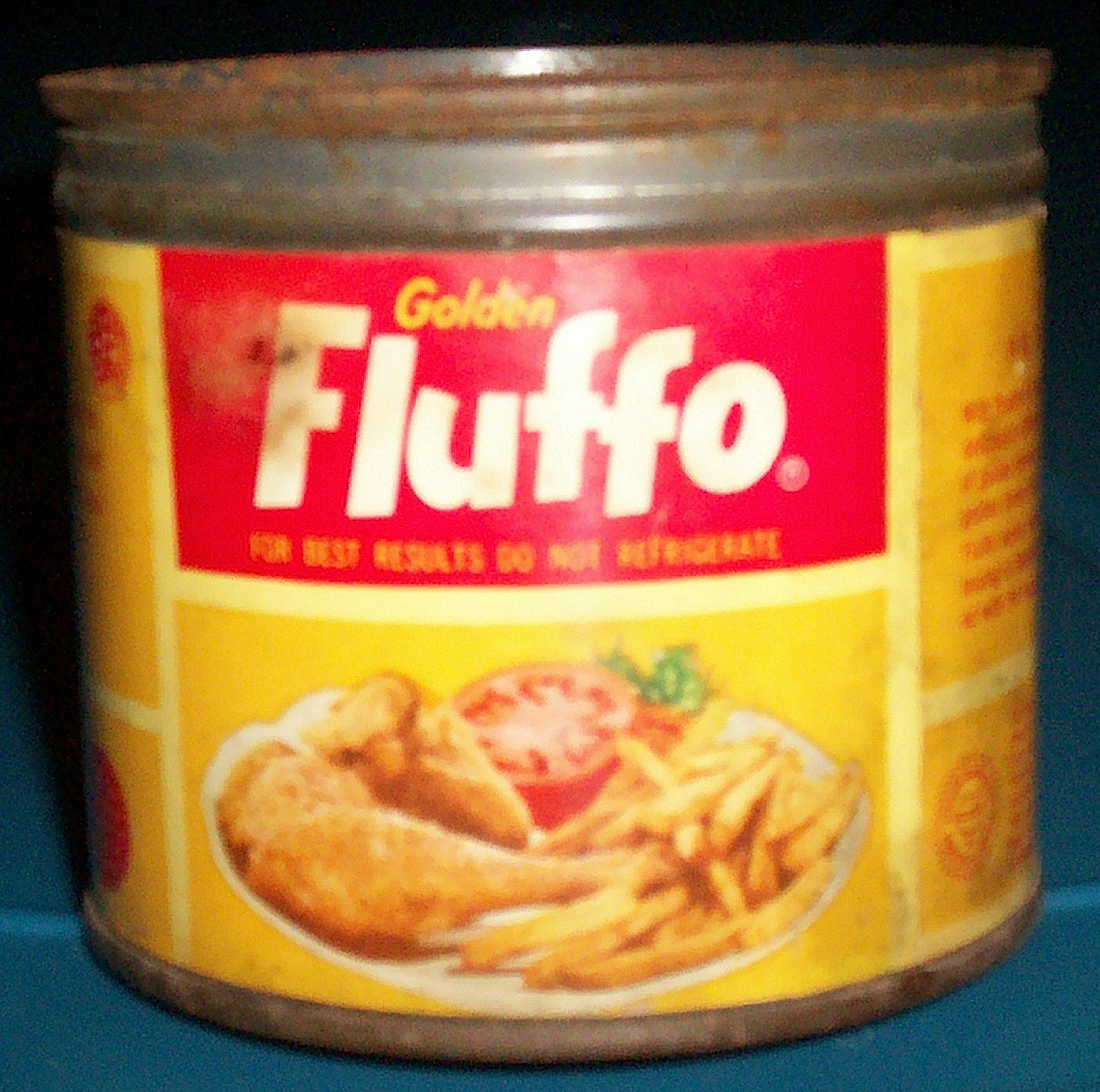This is an up-close photograph of a very old, short, and stubby metal can with a highly rusted top and bottom rim, indicating its age. The can features a yellow label with a prominent red rectangle displaying the brand name "Golden Fluffo" in white letters, and beneath, it states, "For best results, do not refrigerate." The label includes an illustration depicting a platter with pieces of fried chicken legs, possibly wings or a breast, alongside a half tomato, a few leaves of lettuce, and a generous serving of golden-brown fries. The can, positioned on a blue surface, has a black, slightly blurry background due to poor lighting. The design is accented by additional yellow panels on either side, which likely contain nutritional information and ingredients, separated by white lines.